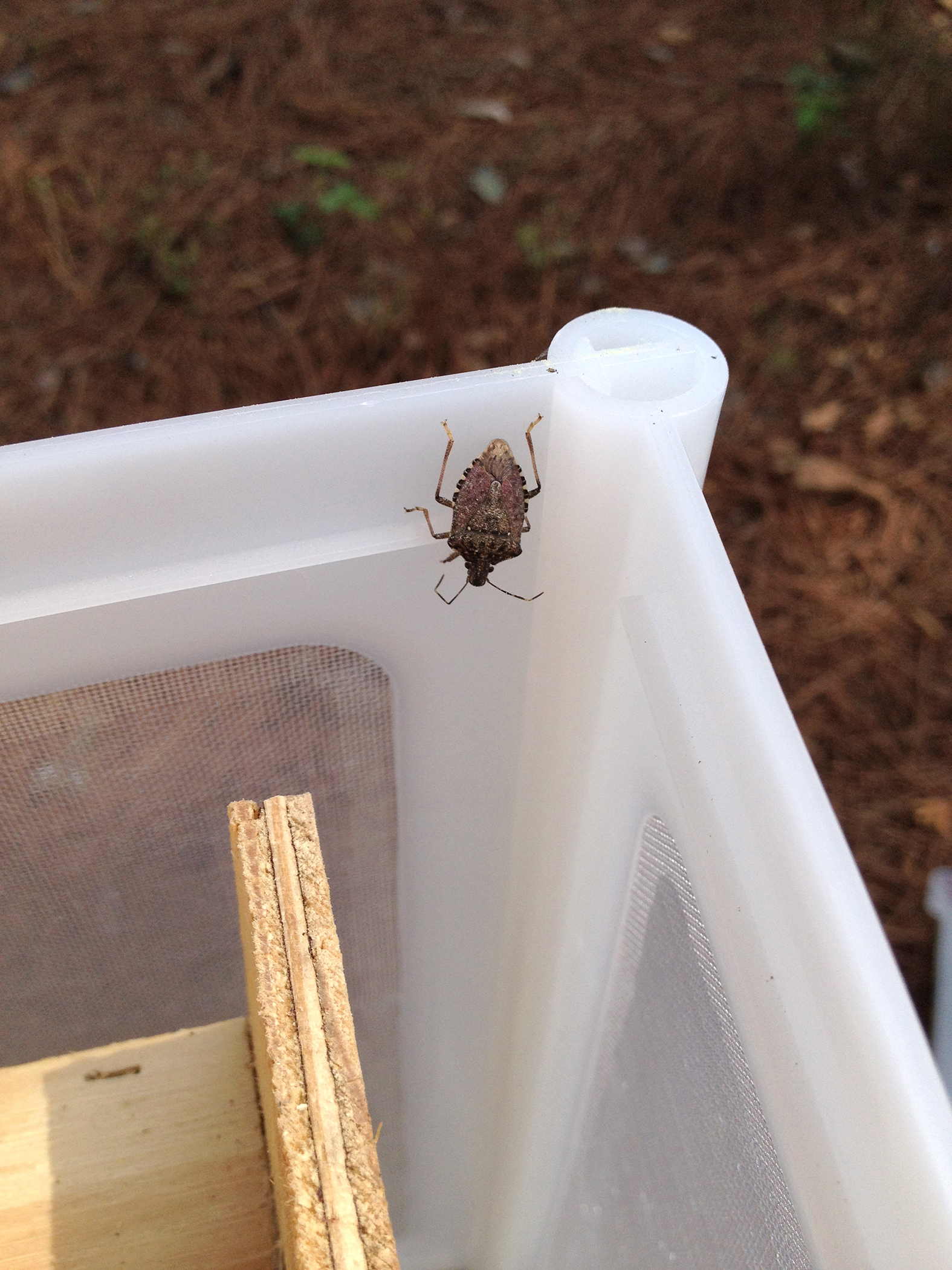This image captures a detailed portrait-mode close-up of a brown stink bug, characterized by its typical black head, positioned in the upper right corner of a milky white plastic container. The container features transparent mesh sides and houses two intersecting pieces of wood: a vertical piece of composite board and a horizontal piece resembling a 2x4 at the left-hand corner. Surrounding the container are earthy, brown mulch with a few green vegetation sprouting through, giving a naturalistic touch to the scene. The background, resembling a forest floor with wood chips and dried grass, completes the outdoor setting of this intriguing moment.